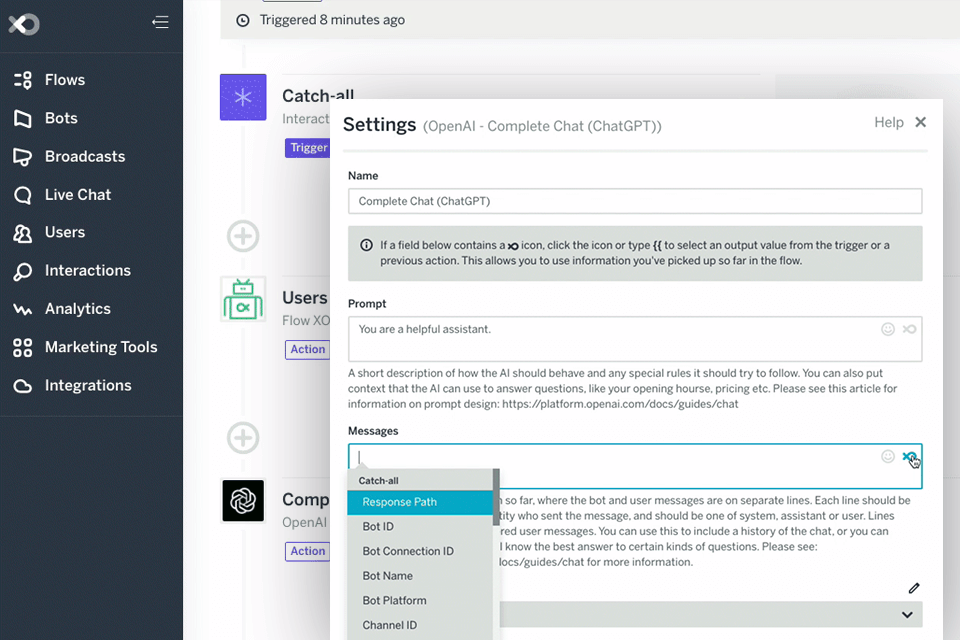A screenshot showcasing the ChatGPT interface from OpenAI is seen in the foreground, partially obscuring the background. The open ChatGPT page prominently displays options for downloads and plugins, suggesting it is the download page for ChatGPT. Behind this, there's a blurred view of additional tools and features including "flows," "bots," "broadcast live chat," "user interaction analytics," "marketing tools," and "integrations." These elements imply that the tool encompasses a broad range of functionalities, enhancing standard ChatGPT capabilities. However, due to the obscured view, the complete list of features remains indistinct.